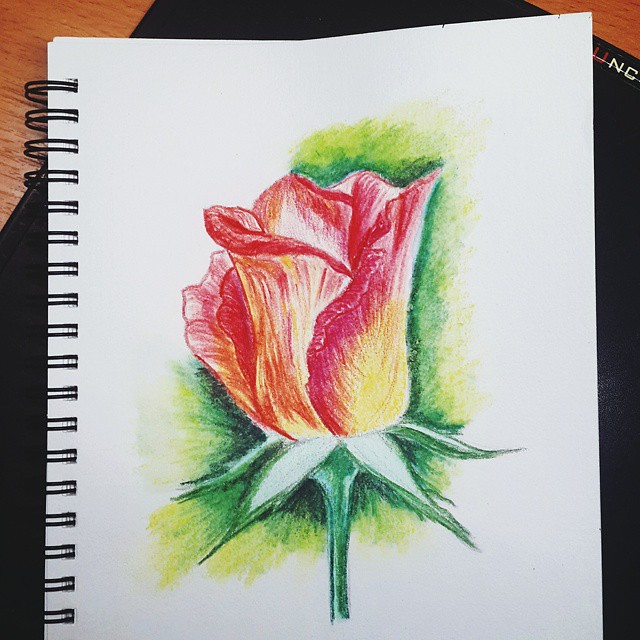This detailed illustration depicts a colorful rose drawn on a white spiral-bound notebook page, which is still attached to the notebook's black spirals. The notebook is placed on a black mat or clipboard, resting on a brown table. In the center of the page, the rose blooms with petals that transition from yellow at the base to red edges, creating a beautiful, lacy effect. The green stem supports the rose along with four dark green leaves that are outlined in a darker green and lightly shaded in the middle. Surrounding the rose is a background that starts with a dark green close to the flower, blending into a lighter green, and eventually fading into yellow about an inch away from the edges of the flower. The upper left corner of the page has no background shading, providing a contrast. Additionally, the top right corner of the page features the letters "UNC," and behind the notebook, there is a black book against the wall, adding an extra layer of depth to the setting.